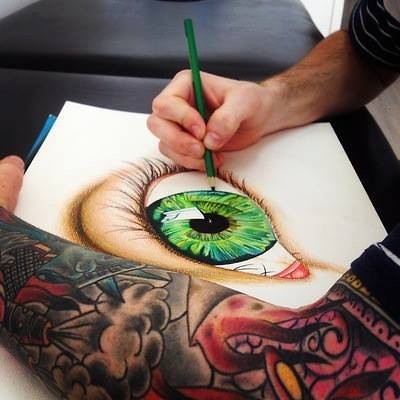In this square photograph, a man with a heavily tattooed left arm, adorned with colorful designs including dark greens, reds, and various indistinct shapes, is holding a sketch pad. The pad contains a detailed color drawing of a large, green-eyed human eye with a realistic green iris, black pupil, and finely rendered eyelashes. Above the eye, sections of skin and eyebrow are visible, meticulously colored in natural tones. The man’s right hand, less tattooed, is actively engaged in drawing with a green colored pencil, which matches the green iris of the eye sketch. The scene is set against a dark background, possibly a black surface or dark leather, which frames the artistic focus. The photograph does not feature the artist’s face, centering attention on the focused creative process of the detailed eye sketch.